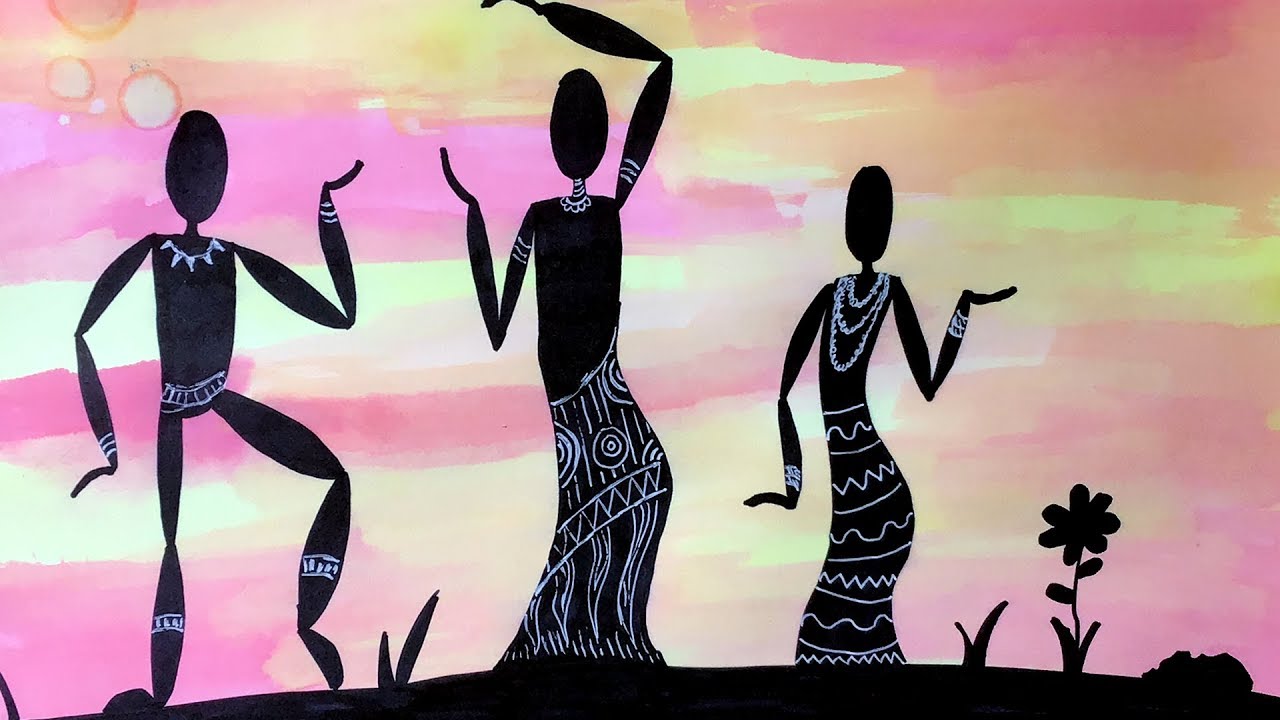This painting features three black silhouetted figures set against a vibrant, multi-colored sky of pink, yellow, orange, and purple hues, resembling a sunset. The style evokes African art, with the figures resembling dancers. The leftmost figure, possibly a man, is featureless and adorned with a white necklace, belt, and anklets. The central figure, likely a woman, has one arm raised toward the sky and is wearing a white choker, bracelets near the shoulders, and a skirt with intricate white patterns. The rightmost figure, also probably a woman, is decorated with three white chains, two bracelets, and a skirt with white designs. The ground is a stark black, contrasting with the colorful sky, and is dotted with silhouettes of a flower and a few plants, adding depth to the scene.